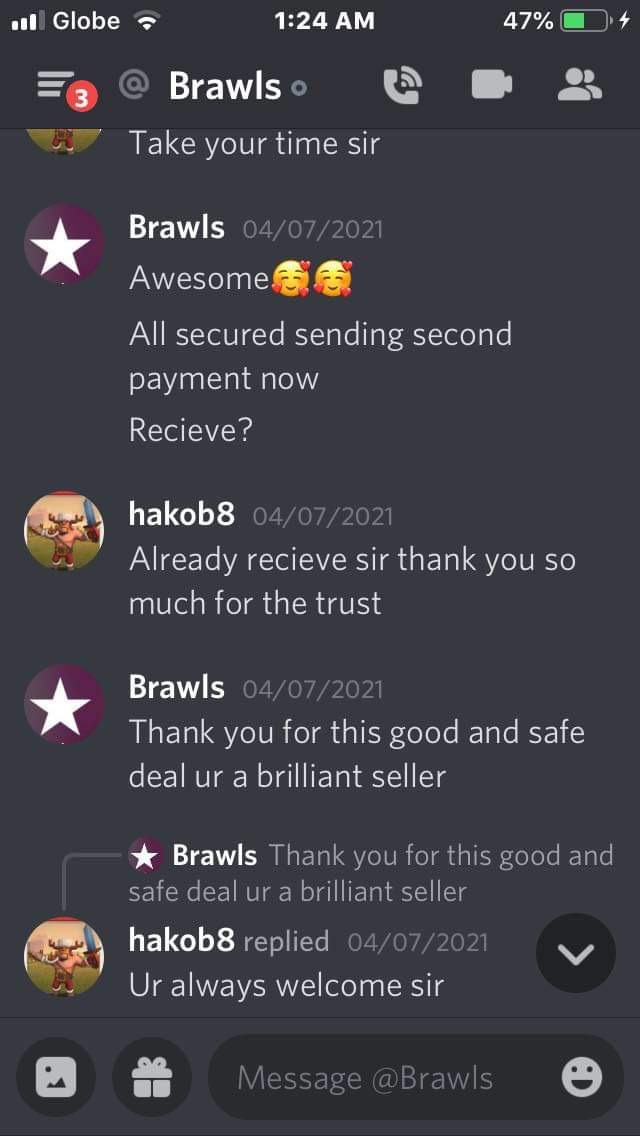This image is a screenshot of a chat room discussion on the Discord messaging app, displayed on a cell phone. Against a grayish-black background, the top indicators show white lettering that says "GLOBE," a Wi-Fi indicator, a cellular signal bar, and a green battery icon at 47%. The timestamp reads 1:24 a.m. 

The chat involves two participants, "@Brawls" and "Hocob8." There's a notification badge with a red "3" next to "@Brawls's" handle, indicating three unread messages. To the right of "@Brawls," there are icons for a phone, video, and group chat.

The conversation begins with someone saying, "Take your time, sir." This is followed by a message from Brawls dated April 7, 2021: "Awesome 😊😊. All secured. Sending second payment now. Received?" 

Hocob8 quickly responds, "Already received, sir. Thank you so much for the trust." 

Brawls replies, "Thank you for this good and safe deal. You are a brilliant seller."

Hocob8 ends the conversation with, "You’re always welcome, sir," spelled "U R always welcome, sir."

At the bottom of the image, there's an option to "Manage @Brawls," and a smiley face along with other symbols.